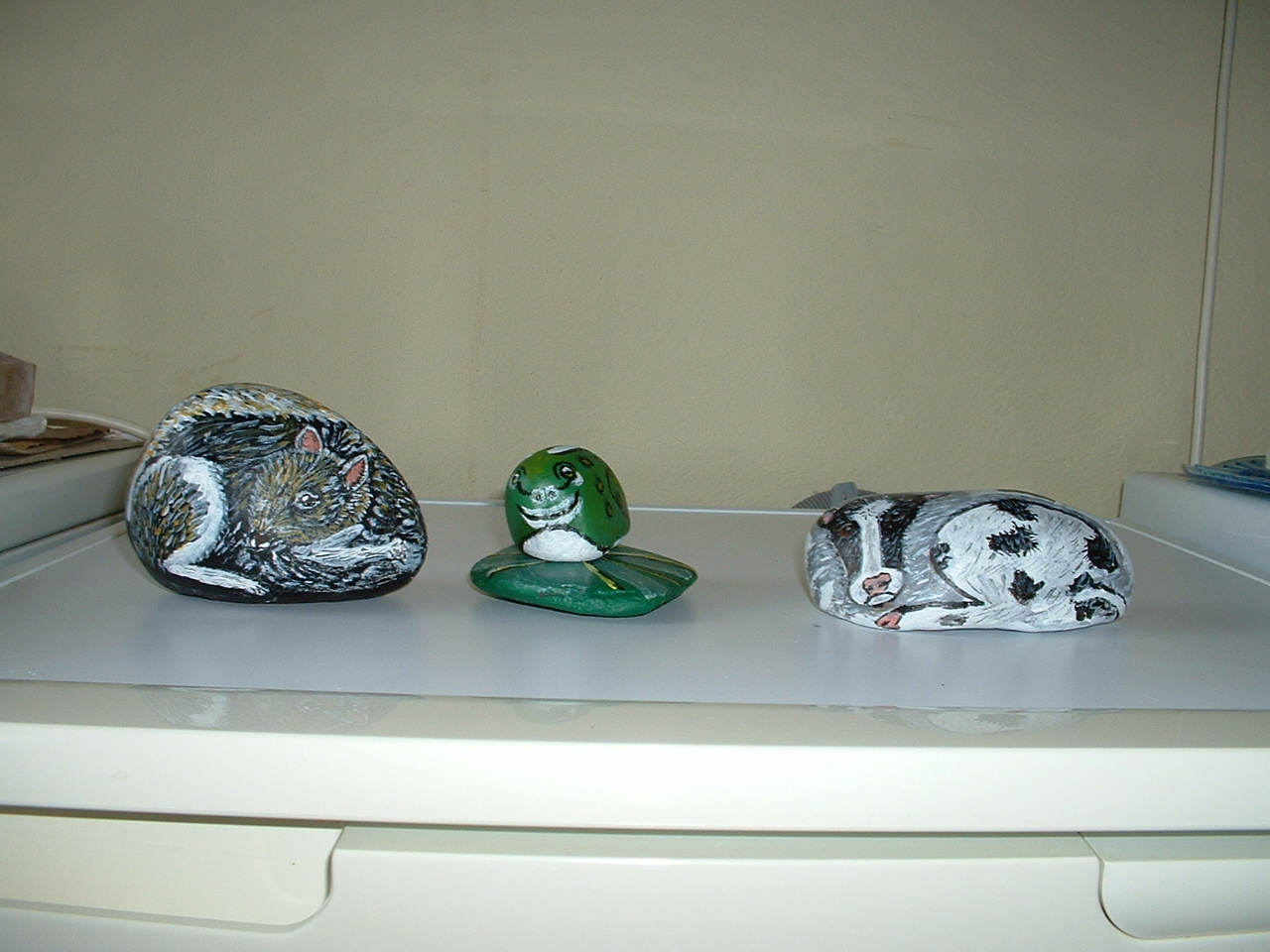In this indoor photograph, a white shelf with a white runner on it is set against an off-white wall. On the runner, three painted rocks are meticulously positioned in a row. On the left, there's an oval-shaped rock featuring the back rear leg and head of a squirrel, painted in gray, white, and brown, as though it's glancing at its leg. In the center is a flat, oval rock painted to resemble a green lily pad, topped with a small, round rock painted green and white with black stripes, possibly mimicking a frog. The rightmost rock is jellybean-shaped and painted to resemble a dog lying down, with its head resting on the left side and its paw curled near its nose. This stone features black, white, and hints of pink for added detail.